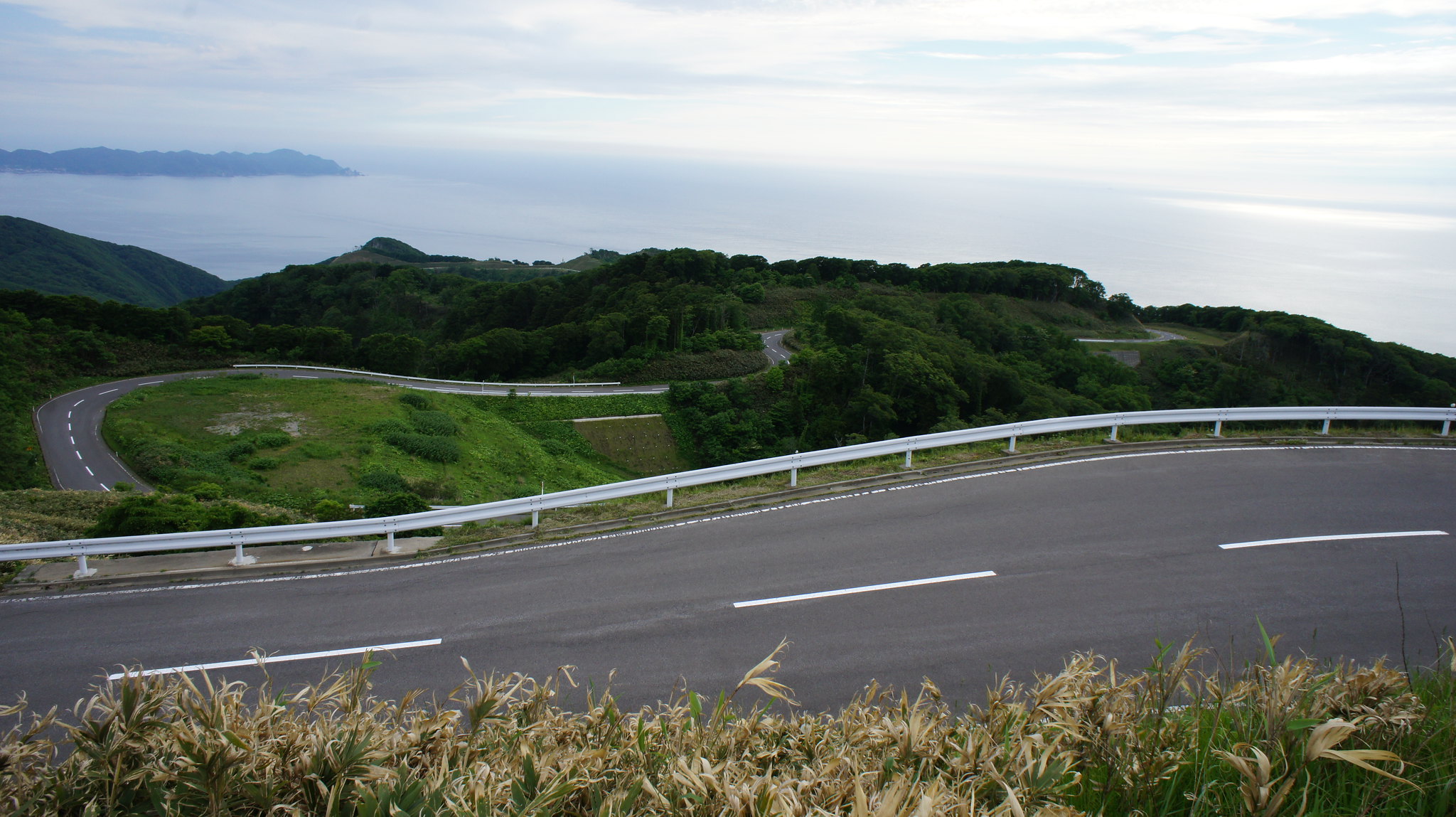This is a detailed color photograph capturing a panoramic scene featuring a two-lane highway snaking through a verdant landscape. In the very foreground, there is a mix of dried beige flowers with green stalks swaying in the wind, set against contrasting green grasses. The road, complete with a guardrail and white dashed lines, lies beyond the patch of foliage. It twists and turns through lush green hills filled with abundant trees and large bushes. The middle of the photograph showcases these trees before giving way to the ocean in the background. The sea, a bluish-gray with a pale blue hue, extends towards the horizon. On the upper left-hand corner, a green piece of land juts into the sea, possibly an island. The sky above is overcast with light, wispy clouds drifting across it. The scene suggests a location with a temperate climate, possibly the UK. The overall ambiance is serene, capturing the interplay between a man-made highway and the serene natural environment around it.